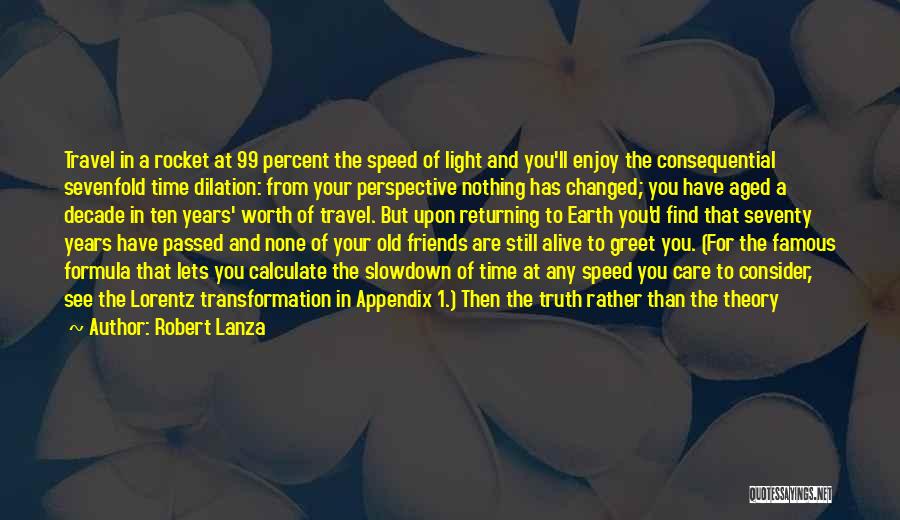The image is a screenshot of a PowerPoint slide featuring a quote by Robert Lanza, with text in yellow centered on a muted, bluish background adorned with five-petaled white flowers. The quote reads: "Travel in a rocket at 99% the speed of light and you'll enjoy the consequential 7-fold time dilation. From your perspective, nothing has changed; you have aged a decade in 10 years worth of travel, but upon returning to Earth, you'd find that 70 years have passed and none of your old friends are still alive to greet you. For the famous formula that lets you calculate the slowdown of time at any speed you care to consider, see the Lorentz Transformation in Appendix 1." The quote is attributed to Robert Lanza, and in the bottom right corner, the text "quotesayings.net" is displayed.